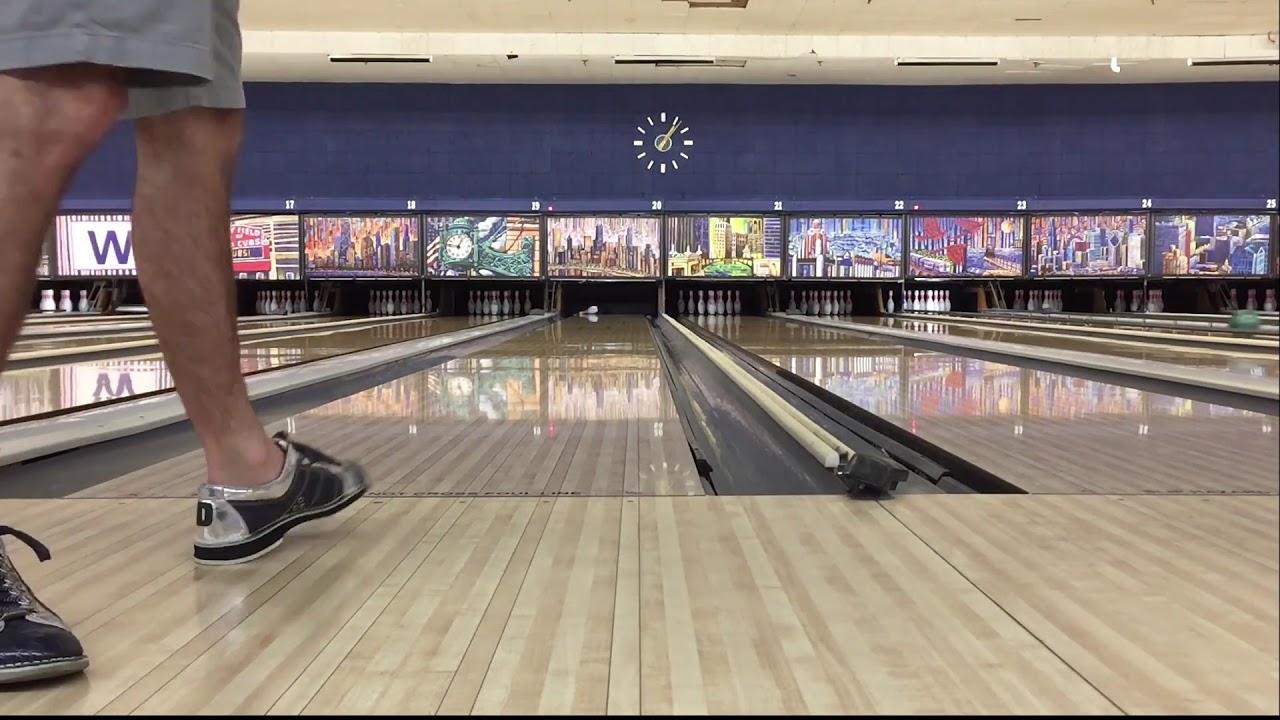This detailed color photograph, taken from a low floor-level perspective in landscape orientation, captures the polished, light brown, and tan paneled wood floor of a bowling alley. The image highlights multiple bowling lanes, with the central lane showing a single bowling pin lying on its side amidst an otherwise pin-clear lane, indicating a recent throw. On the left, a person, wearing gray shorts and black and silver bowling shoes, stands partially visible, with the frame cutting off at their knees. Above the lanes, vibrant cartoon cityscapes adorn the walls, leading up to a solid blue wall featuring a clock with yellow hands and white dash marks as numbers. This striking scene epitomizes photographic representational realism, bringing the lively environment and the motion of the game to life.